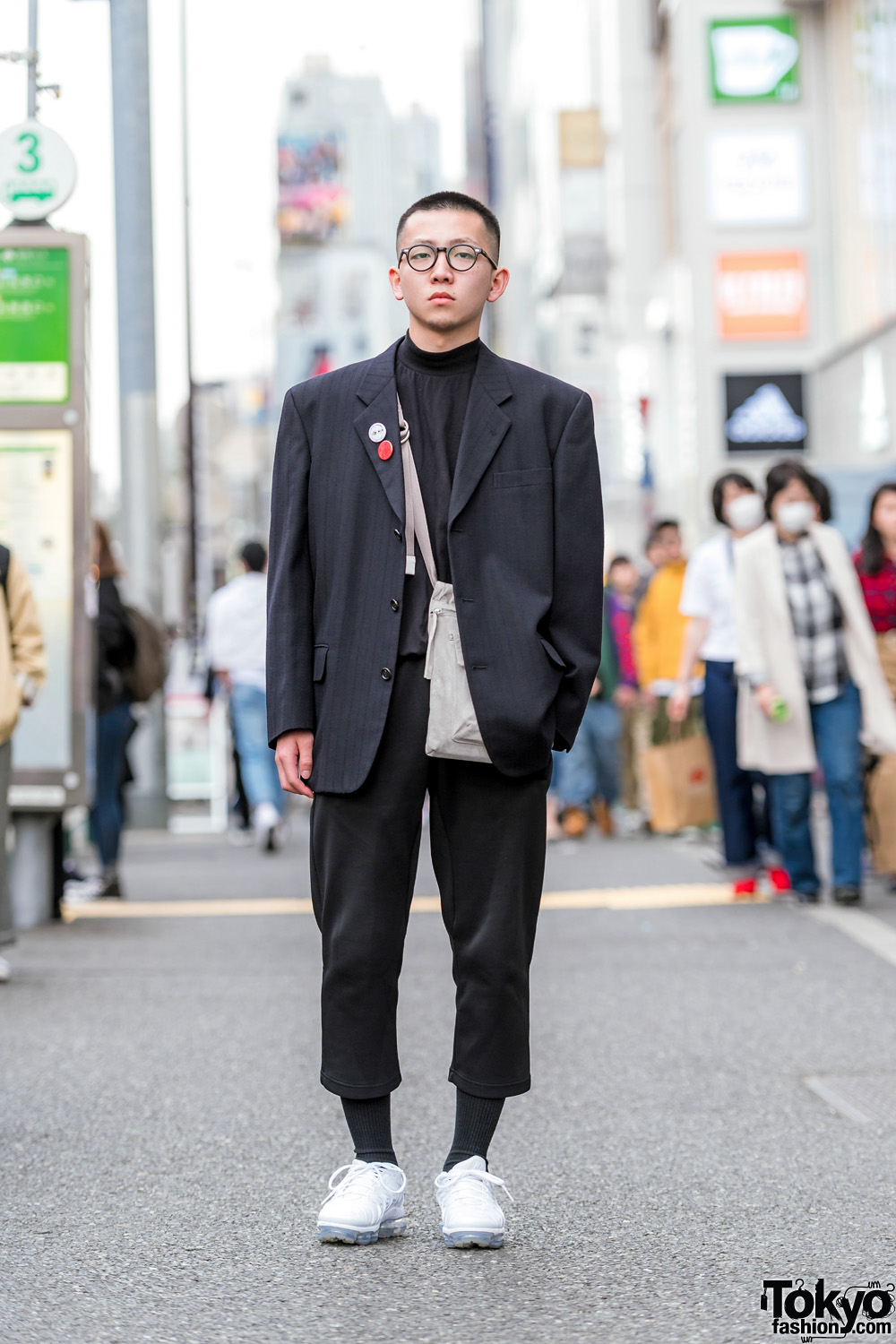The image is a color photograph set in a busy sidewalk area in Japan, with the focal point being a young Asian man. He has a close-cut, military-style haircut and wears round glasses. The man is dressed in a charcoal gray, baggy blazer over a black stand-up collar t-shirt, paired with slightly baggy, ankle-length pants and white tennis shoes with black socks. He has a silver satchel slung across his right shoulder and tucked behind the jacket. His left hand is casually placed in his pocket. Surrounding him are blurry high-rise buildings, various signs with glimpses of green, and several people, predominantly on the right side, some wearing face masks. A blurred Adidas logo is faintly visible in the backdrop. In the bottom right corner of the image, the text "TokyoFashion.com" is displayed in black.